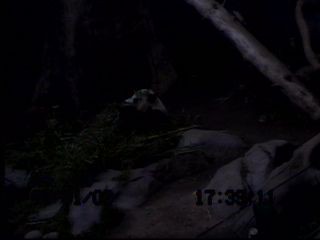The photograph, taken at 17:38:11, captures a nighttime scene through a possibly security or nature cam. The image is quite dark, with the far background being a solid pitch black indicating it was taken after sunset. The most prominent feature is a cluster of brown rocks stretching diagonally from the center to the lower left of the frame. Atop the rocks, there is a white creature, its details obscured by the darkness. The top right corner of the image is intersected by a tree branch that extends towards the middle. Imposed onto the image are several unreadable numbers, except for "1/0" hinting at a partial date on the left and a clearer timestamp on the right. The overall scene presents a somewhat eerie atmosphere, enhanced by the obscure visibility and dim lighting.